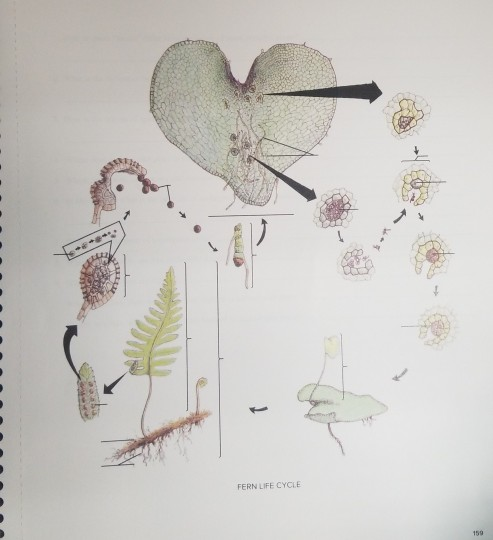This image is a detailed diagram of the fern life cycle, drawn on a notebook page. The notebook ridges are visible at the bottom left. The central feature is a greenish-gray, heart-like shape at the top middle, with dark blue arrows extending to the right and bottom. This heart-like object has black cracks and hair growing from its center. To the right, there's a succession of cell-like formations: yellow ones leading to purple ones, connecting via arrows. 

At the bottom right, a small light green shape, reminiscent of a cucumber, is connected by an arrow to the left, directing to an illustration of fern roots and a sprouting fern plant with a green leaf bearing little spikes. Another light green structure nearby has an arrow pointing leftward. Above these, there's a reddish-purple oval shape with a line at the bottom, followed by another similar reddish-purple shape.

Throughout the diagram, multiple arrows indicate the progression of different stages, highlighted by purple, light green, and yellow hues. The specific sequence shows various cellular structures transforming and leading up to the recognizable fern leaf. The diagram is labeled "Fern Life Cycle" at the bottom, with the number 159 noted at the bottom right.